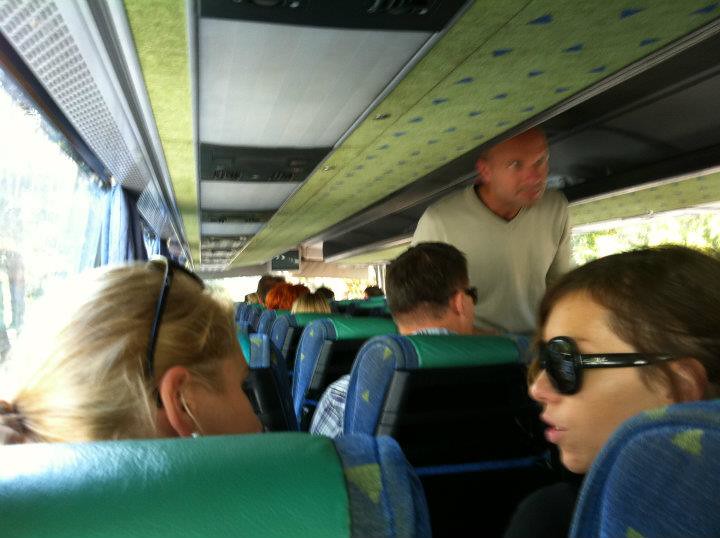The image captures the scene inside a bus from a perspective directly behind two female passengers. The focus is on these two women: one with blonde hair, pulled back, and glasses resting on top of her head; the other with brown hair, also pulled back, wearing dark black sunglasses. They are engaged in a conversation facing each other. Both are seated on plush blue and green seats. The interior of the bus features a ceiling adorned with lime green and black stripes, adding to the vibrancy. To the right of these women, a man in a light green, long-sleeved sweater is making his way down the aisle, his bald head clearly visible. Further ahead, various passengers of different genders and hair colors can be seen sitting, including a man with short dark hair and sunglasses. The entire scene is enveloped in the cozy, multi-colored interior of the bus, with rows of similar blue and green seats continuing towards the front.